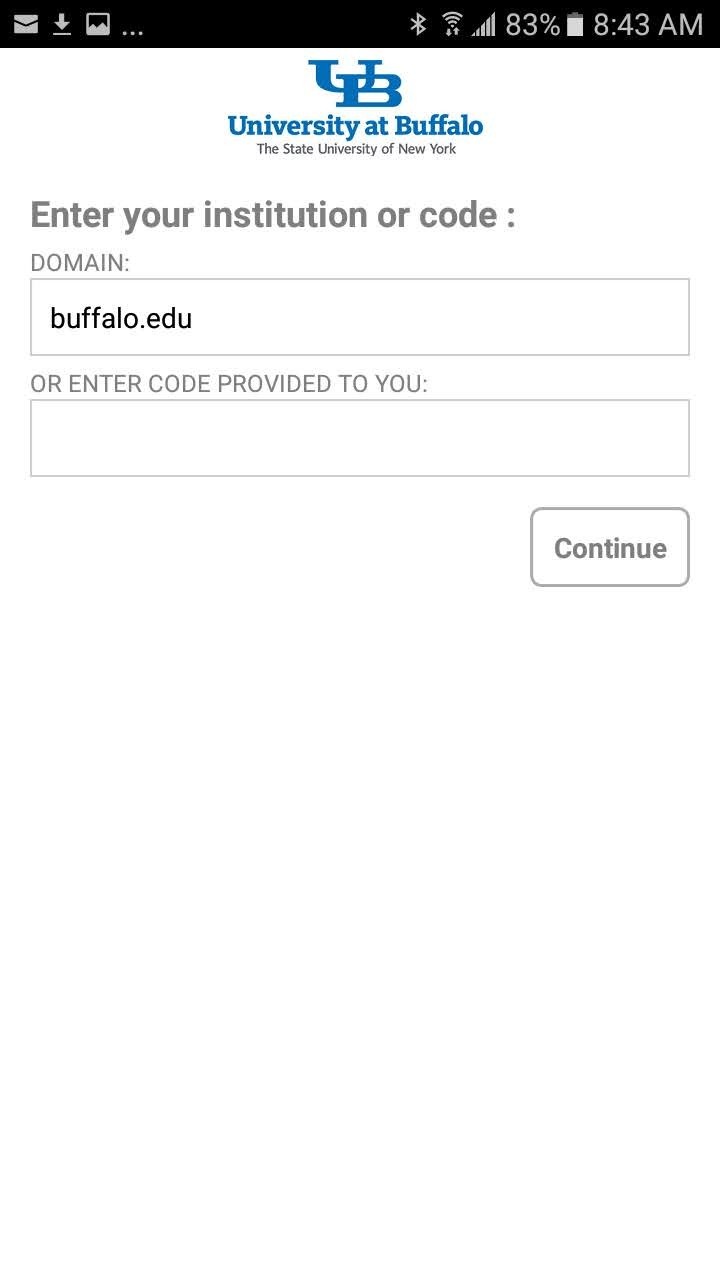This image showcases a cropped screenshot from a mobile device displaying a portion of a University at Buffalo (State University of New York) login or registration page. The prominent elements include the University's logo, represented by a stylized 'UB', positioned near the top of the screen. Below the logo, users are presented with two text fields. The first text field is designated for inputting a domain, where someone has entered "buffalo.edu". The second text field offers an alternative input method, allowing users to enter a code provided to them.

Beneath these input fields lies a prominently placed "Continue" button. The rest of the screen is mostly filled with white space, suggesting a clean and unembellished interface likely meant for simplicity and focus on the task. 

At the very top of the image, the phone's notification bar reveals various status indicators: the current time is 8:43 AM, the battery is charged to 83%, and the device shows full network bars with a strong Wi-Fi connection. Bluetooth is also enabled and connected. The notification icons indicate unread mail, a recent download, and a freshly taken screenshot. This screenshot portrays a succinct and functional user interface, possibly related to logging in with a university email or registering for a service affiliated with the university.